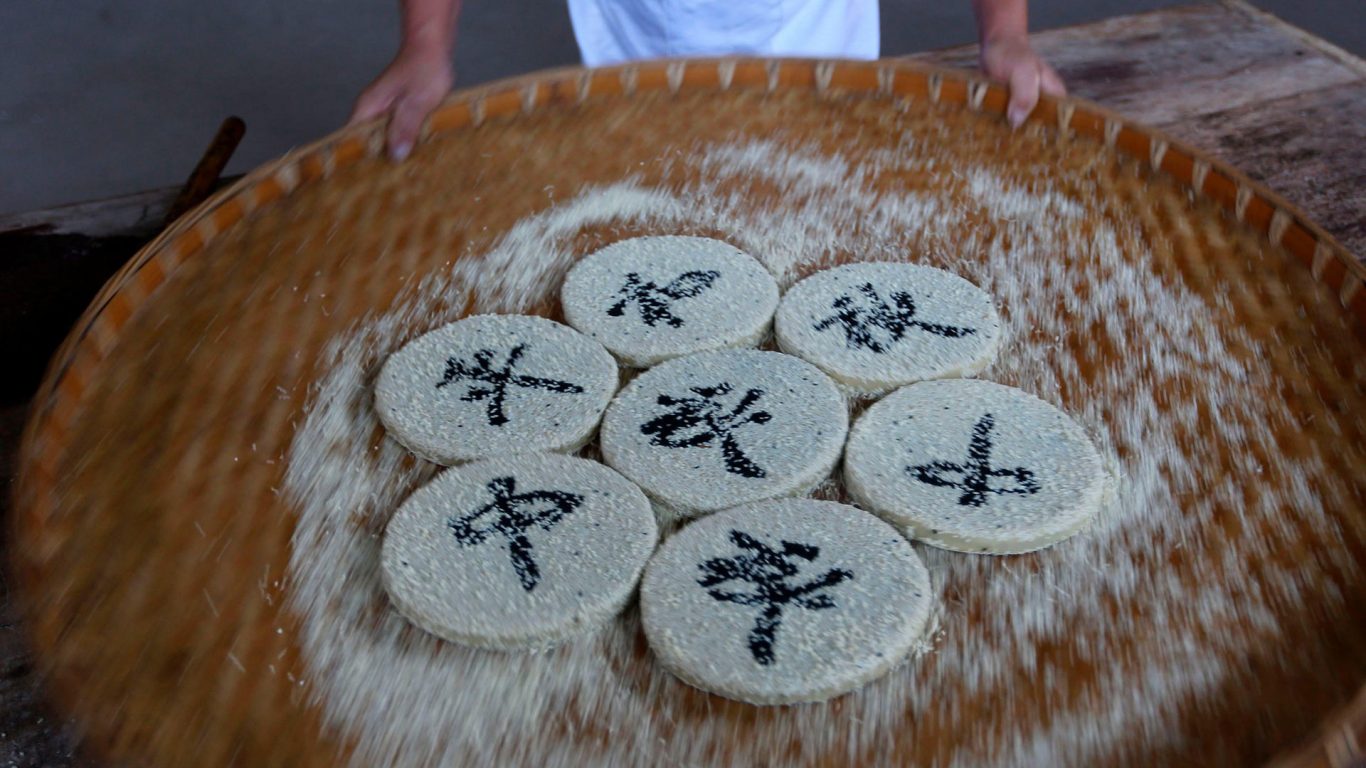This image captures a traditional East Asian culinary scene, focusing on the preparation of what appear to be rice cakes or similar items. Each round, flattened disc is adorned with intricate black patterns or Chinese characters, possibly indicating decoration or branding. The rice cakes are arranged on a large, round, woven bamboo tray, which is being held by a person whose arms and partial torso are visible. The person is wearing a white shirt, suggesting their involvement in the culinary preparation. The image is an action shot, with the background blurred to draw attention to the tray and its contents. The detailed patterns on the rice cakes stand out vividly, signaling a demonstration or traditional cooking process. Despite the blur, the essence of traditional East Asian food culture is palpable, making the viewer almost taste the delicious-looking rice cakes.